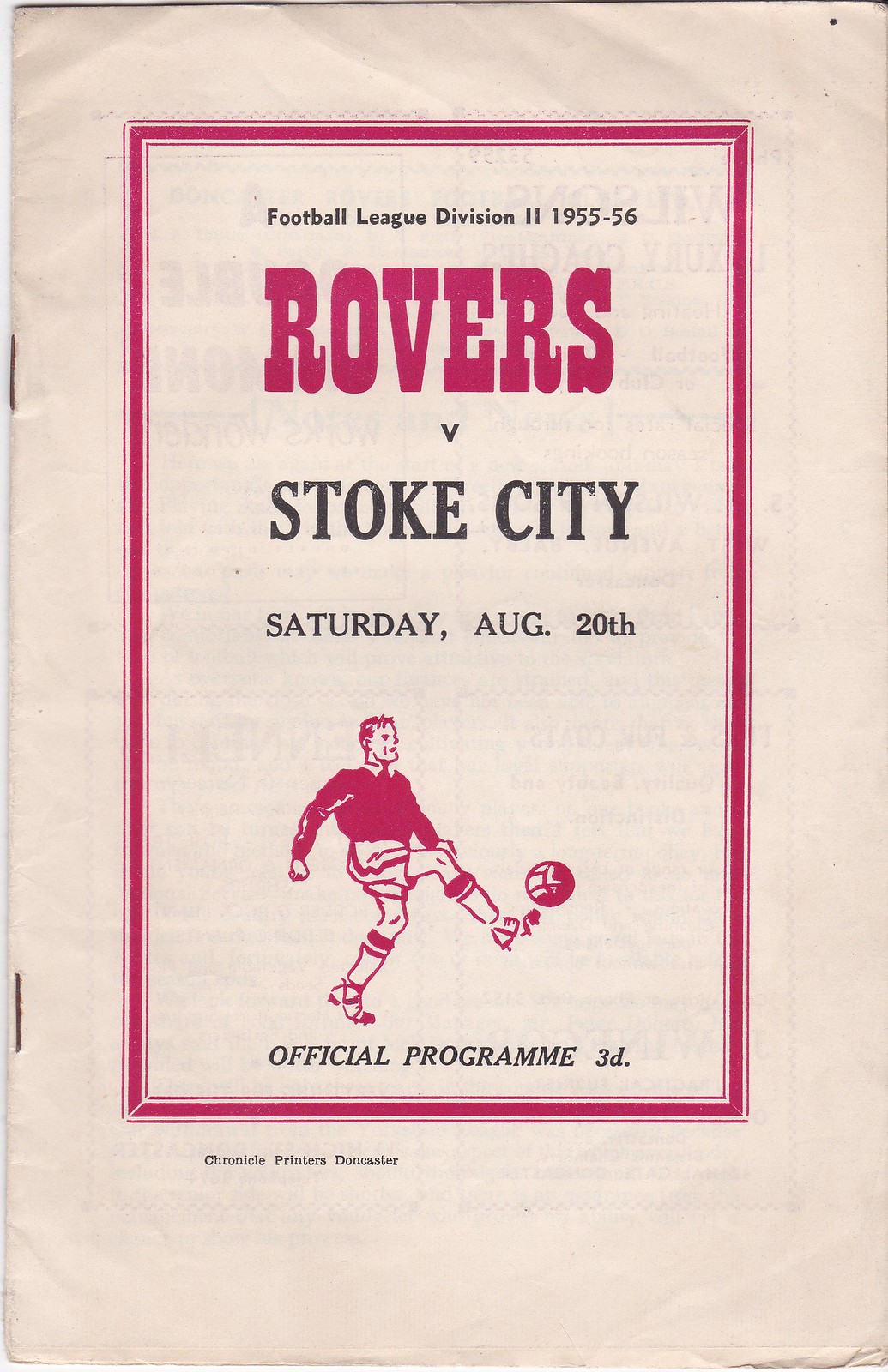This is a vintage program cover from a soccer match, specifically a creamy, aged paper with noticeable browning, wrinkles, and chipping, indicative of its age from the mid-1950s. The cover is bordered by a pink rectangle. At the top, in bold black letters, it reads "Football League Division II, 1955-56." Just below, "Rovers" is prominently displayed in large pink letters, followed by "V. Stoke City" in black bold letters, indicating the teams. The date, "Saturday, Aug. 20th," is written in smaller black text. Centrally, there's a pink illustration of a man in a red shirt and shorts kicking a soccer ball, adding a dynamic element to the design. At the bottom, it states "Official Program 3D" in black text, denoting the program's cost. Additionally, fine print at the very bottom credits "Chronicle Printers Doncaster" with its production.